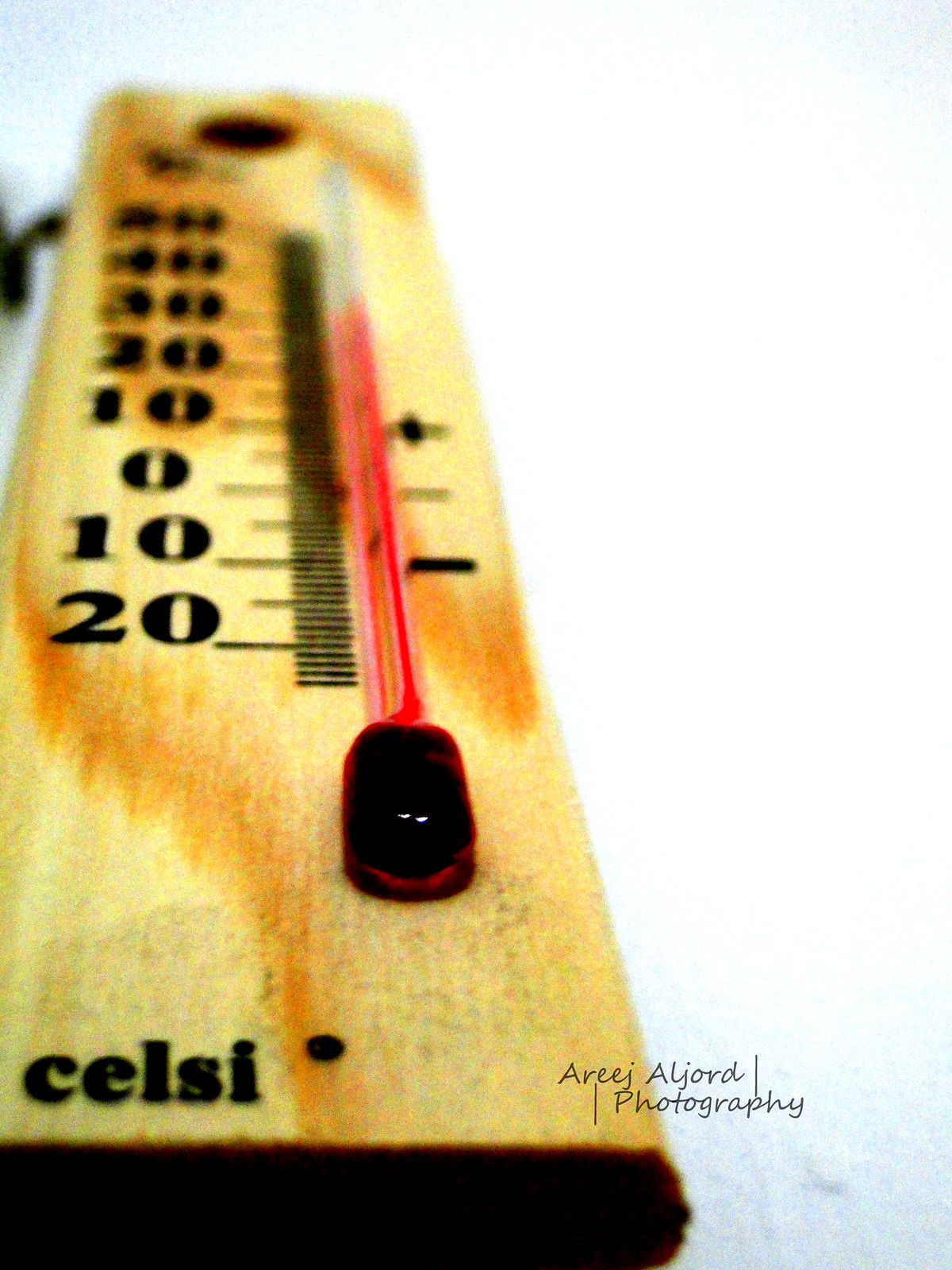This is a close-up image of a wall thermometer crafted from a long, rectangular piece of wood. The wood has a very light pine finish, adorned with subtle, orange-tinted patterns that add a touch of rustic charm. The thermometer is designed for indoor use, measuring ambient room temperature. Black ink temperature markings are clearly visible, ranging from -10 to 50 degrees Celsius, with additional markings for -0, 0, 10, 20, 30, and 40 degrees. The red mercury-like gauge, encapsulated in a glass tube, runs alongside these markings, indicating the current temperature. At the bottom of the thermometer, the word "CELSI" is written in black, presumably indicating the Celsius scale used for measurement.